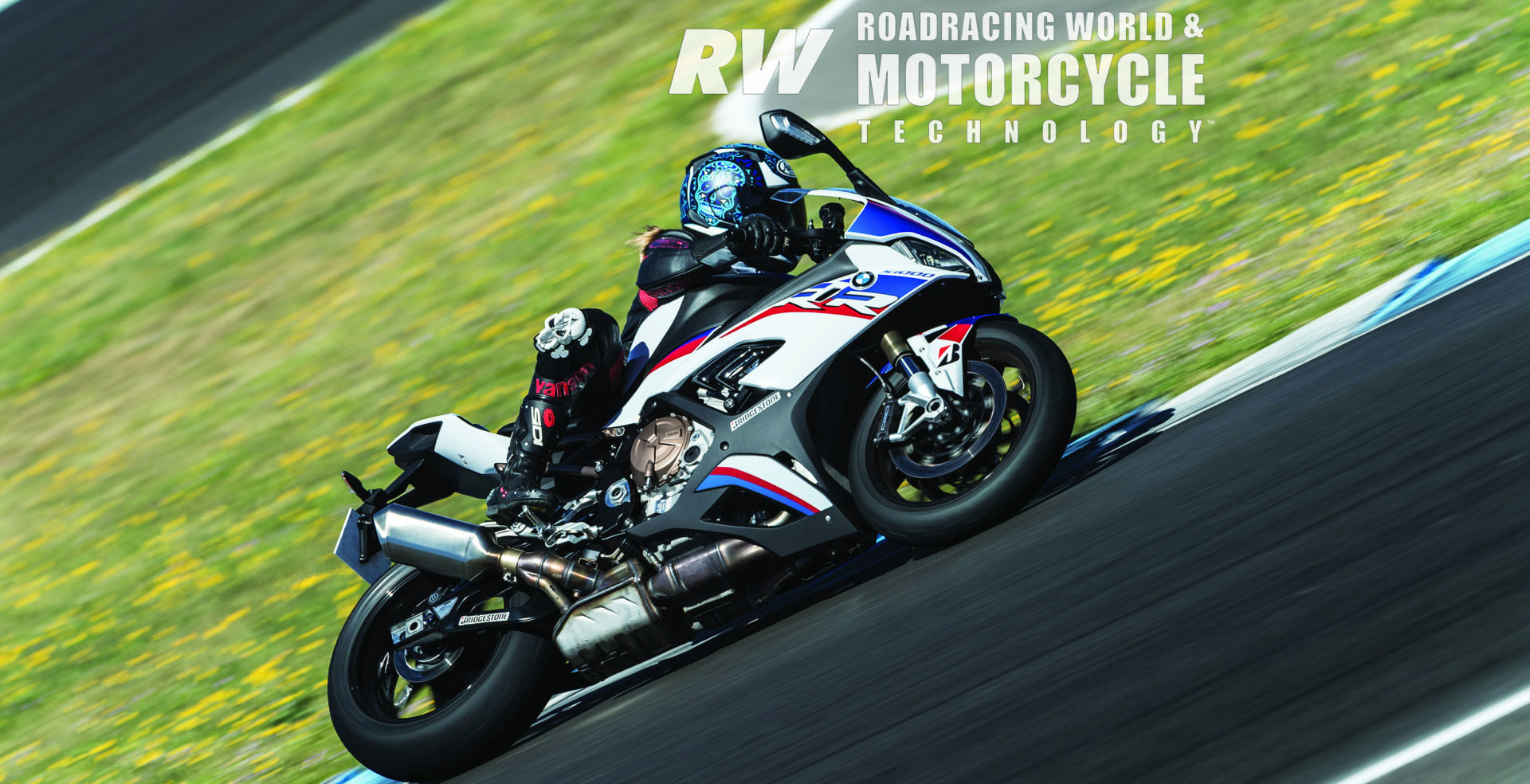In this dynamic advertisement for Road Racing World and Motorcycle Technology, a rider expertly leans into a turn on a sleek sports motorcycle adorned with striking white, red, and blue stripes. The motorbike, with its smooth tyres and prominent exhaust, is seen tilting sharply, almost skimming the ground, emphasizing the high-speed action. The rider is equipped with a black and blue helmet, a black and red suit, and essential protective gear, including knee pads for optimal safety. The image captures the blur of the black, smooth pavement and the streaks of greenery and dandelions in the background, highlighting the incredible speed of the scene. Bold white lettering spells out "RW" and "Road Racing World Motorcycle Technology" across the frame, reinforcing the intensity and precision of this thrilling road racing moment.